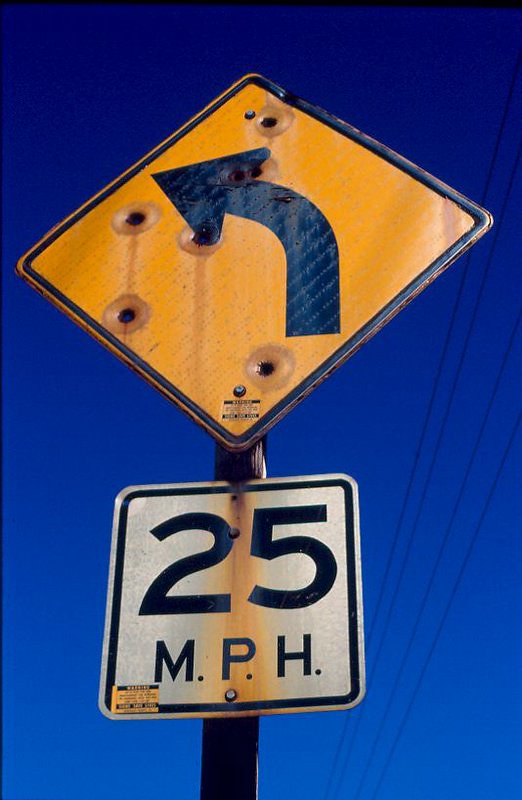This weatherworn road sign warns drivers of a sharp left-hand turn ahead, urging them to reduce their speed to 25 miles per hour. It has sustained significant damage over time; five bullet holes punctuate its surface—a shot at the top, another at the bottom, two on the left side, and one nearly at the center. These impacts have caused noticeable deformations, with the paint around them discolored and marred by rust. The top portion of the sign has corroded significantly, imposing on the secondary sign beneath it. The scene is set against a backdrop of a deep, dark blue sky, unmarred by clouds. Adding to the composition are power lines that run parallel to the sign on the right, extending beyond the field of view.